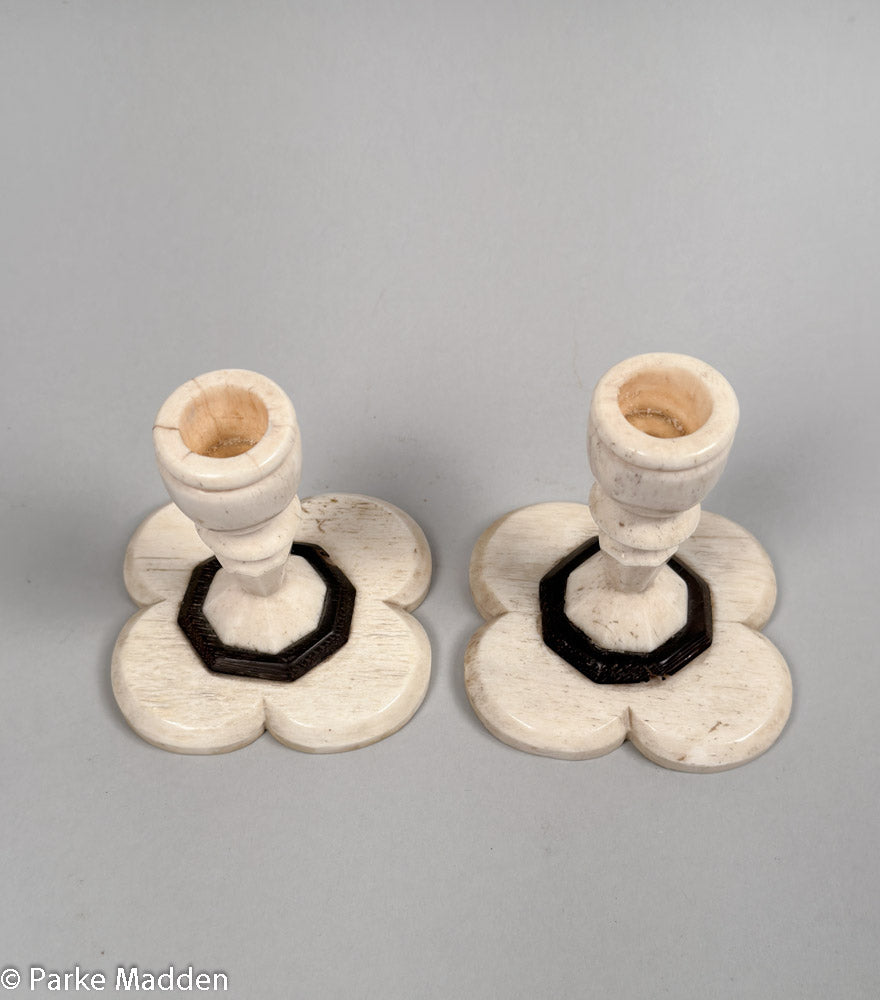The image shows two intricately designed objects, which appear to be candle holders, possibly carved from ivory. Each holder has a delicate, flower-like base resembling a four-leaf clover, but with round sections that converge. The base houses a near-black, marble-like circular structure at the center. Rising from this structure is a hollow, protruding section forming the main body of the holders. The color of the candle holders is predominantly a creamy brownish-gray. The background is plain gray, intensifying the focus on the objects. In the lower left corner of the image, there's white text that reads "© Parke Madden" in precise lettering.